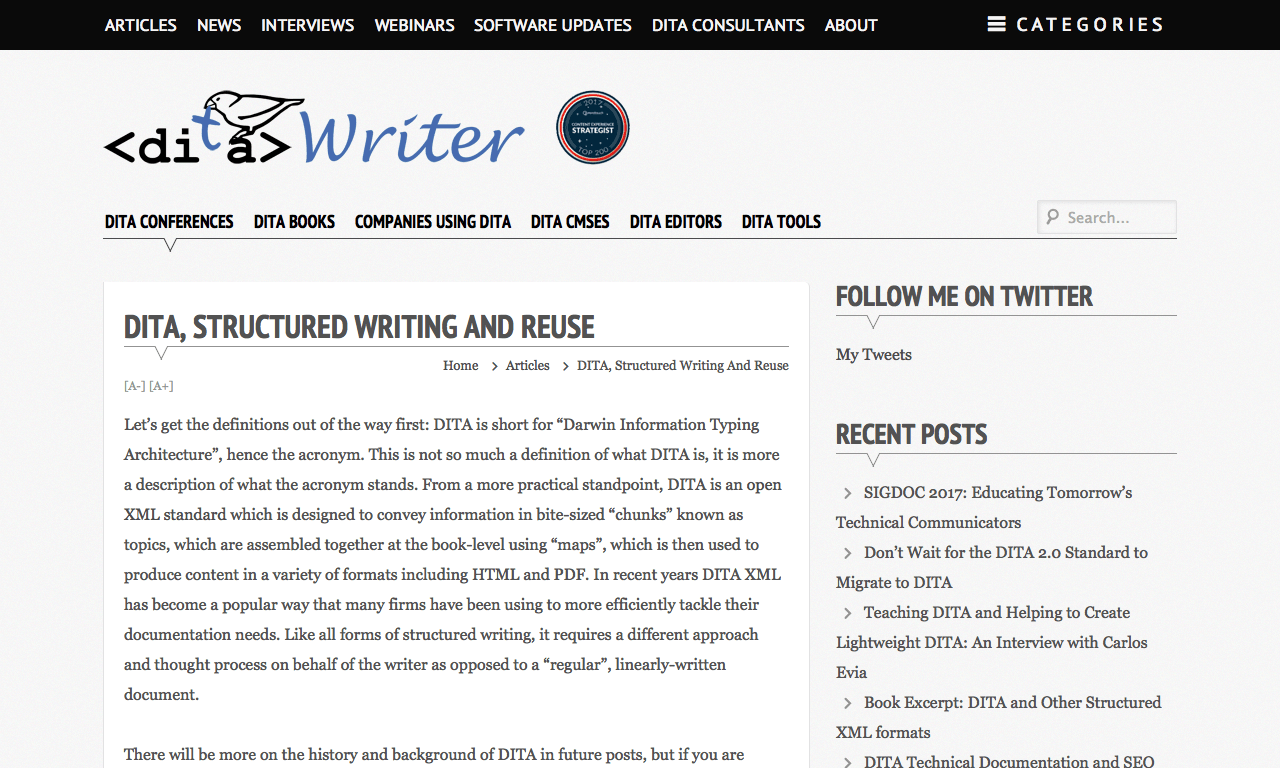The image is a detailed screenshot of a web page featuring a black menu bar with white, capitalized text displaying various menu options. These options include "ARTICLES," "NEWS," "INTERVIEWS," "WEBINARS," "SOFTWARE UPDATES," "DITA," "CONSULTANTS," "ABOUT," and a three-line menu icon labeled "CATEGORIES." The rest of the website has a light gray background, while the main content area consists of a white background with black text.

The blog title, "DITA Writer," prominently appears at the top, with "DITA" stylized uniquely. The word "DITA" is formatted with a left-pointing arrow before the letter "D" and a right-pointing arrow after the "A," all in black. The letters "D," "I," and "T" are in black, with "T" being placed by the beak of a black-outlined bird perched on the black "A." Adjacent to this, the word "Writer" is inscribed in blue script.

Beneath the main menu, several submenus are visible, presenting options such as "DITA Conferences," "DITA Books," "Companies Using DITA," "DITA CMSes," "DITA Editors," and "DITA Tools." The "DITA Conferences" submenu is selected, leading to an article titled "DITA Structured Writing and Reuse."